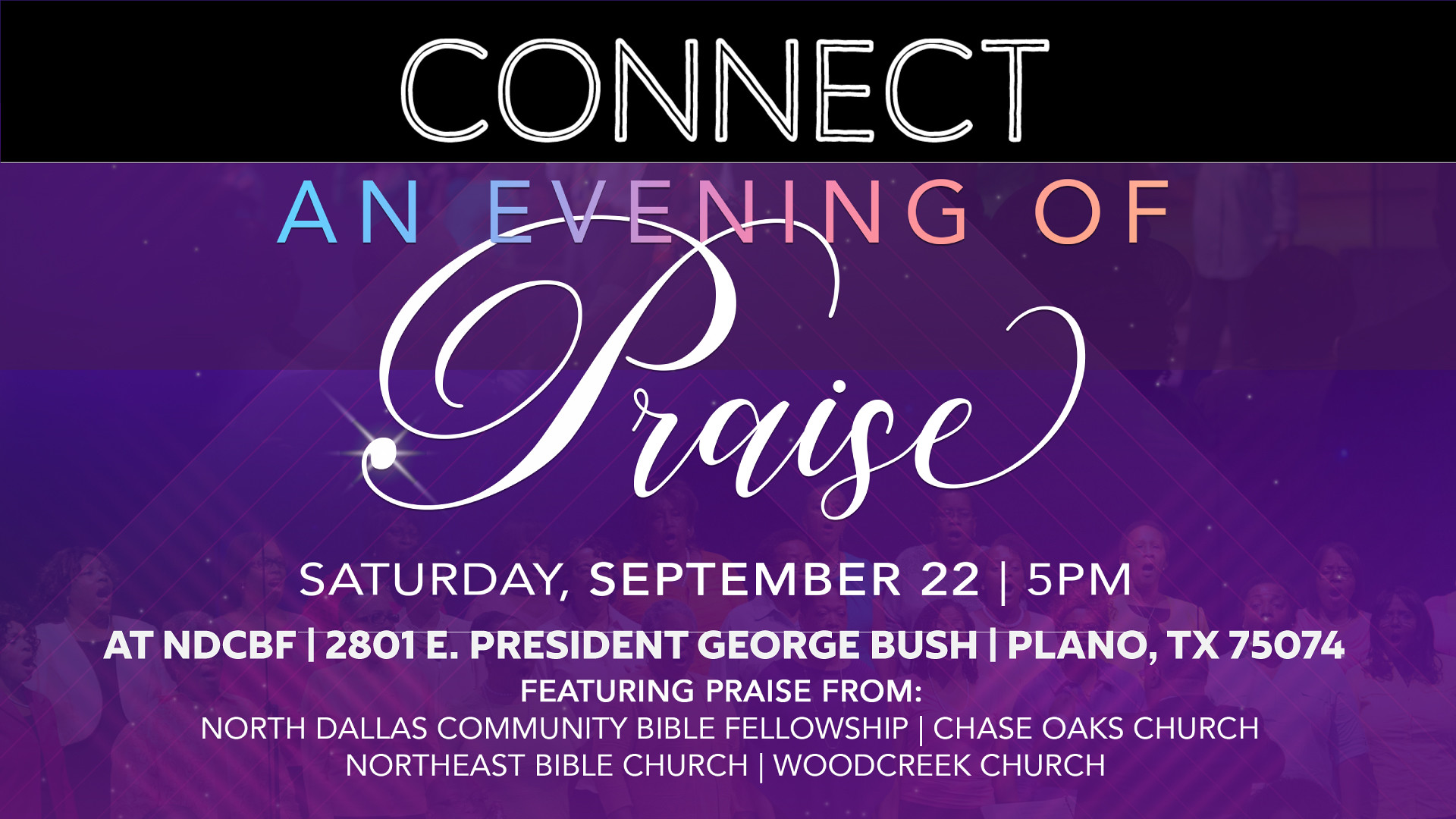JOIN US FOR AN EVENING OF PRAISE

SATURDAY, SEPTEMBER 22ND, 5PM AT NDCBF 
2801 EAST PRESIDENT GEORGE BUSH, PLANO, TEXAS 75074

FEATURING PRAISE FROM 
NORTH DALLAS COMMUNITY BIBLE FELLOWSHIP, CHASE OAKS CHURCH, NORTHEAST BIBLE CHURCH, WOOD CREEK CHURCH

Experience a night of worship and celebration with voices raised in harmony. This vibrant advertisement showcases a black header with "CONNECT" written in bold white capital letters, setting the tone for an uplifting and communal event. The rest of the text, standing out elegantly against various shades of purple, some light and some dark, provides all the essential details, ensuring it captures your attention.

Highlighted against the intricate background of purple and blues, you’ll see a choir of individuals uniting in song, creating a welcoming and spiritual ambiance. The colors – blending blue, orange, pink, and white fonts – add to the dynamic and engaging design, guiding you through the evening's agenda effortlessly.

Don't miss this incredible opportunity to connect with your community and experience the power of praise. Be there at North Dallas Community Bible Fellowship, and let the music lift your spirit.